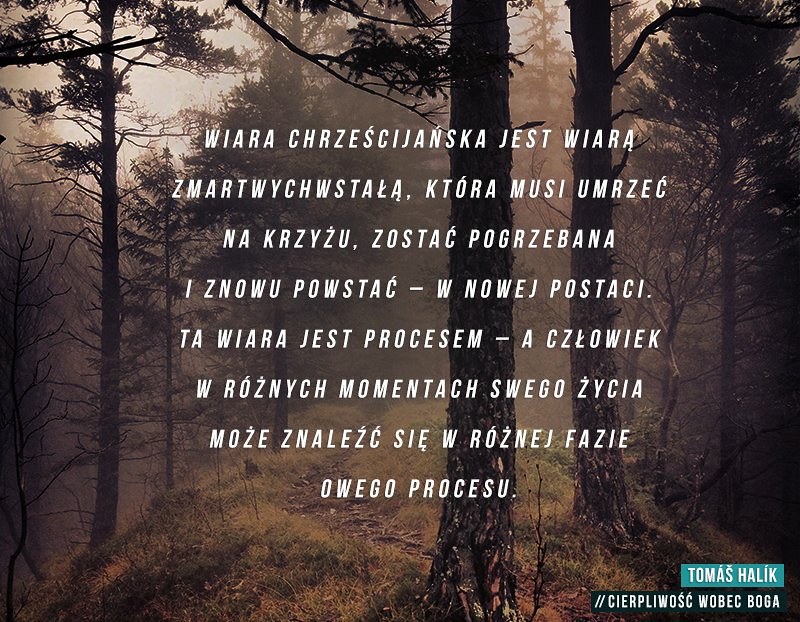This image features a muted, sepia-toned forest with approximately eight to ten trees, some grass, and a narrow path. Superimposed over the forest are eight lines of white text in a different language. In the lower right corner, the name "Tomas Halik" is prominently displayed on a blue banner, with a longer, thinner black banner containing additional white text underneath.